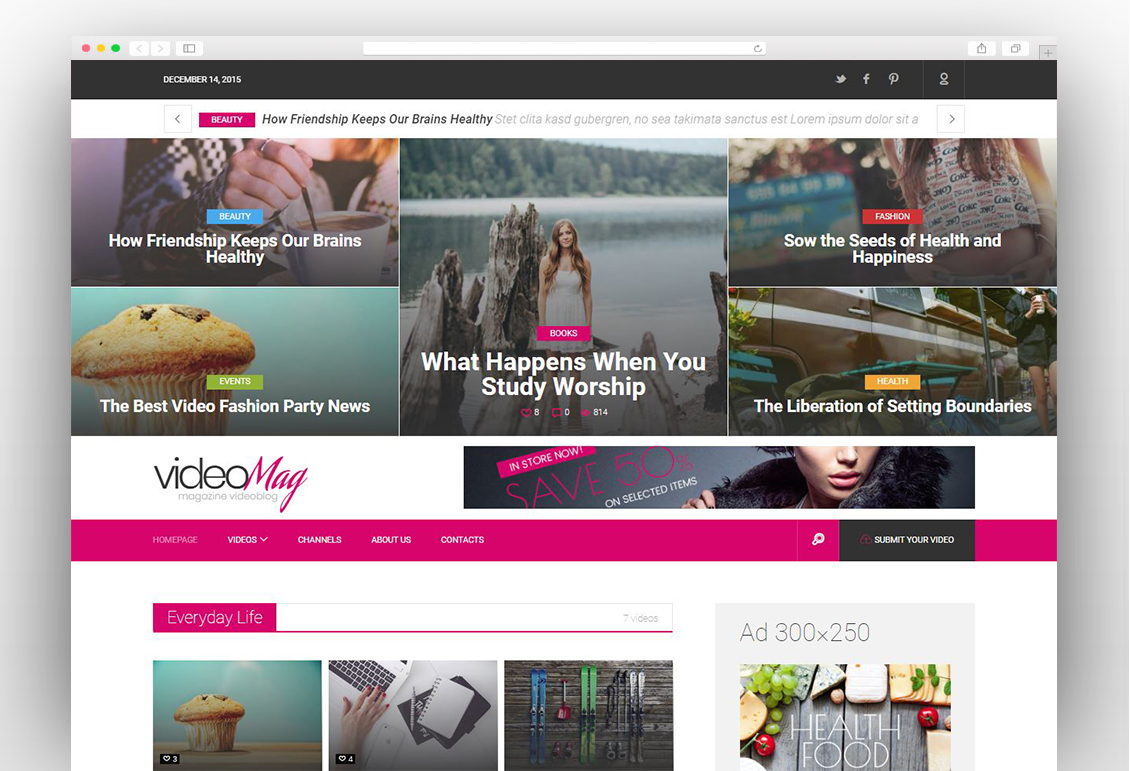This screenshot captures a detailed snapshot of a website interface. In the upper left corner, there are three circular indicators colored red, yellow, and green, followed by a left-facing arrow and a right-pointing arrow. Adjacent to these indicators, there is a bar for entering a web address and a home button. In the upper right-hand corner, a plus sign suggests an option for adding a new page.

Directly below, a black bar stretches across the width of the page, featuring the date "December 14, 2015" in white text. To the right of the date, icons for Twitter, Facebook, Pinterest, and a user profile are neatly aligned.

Beneath the black bar, a white bar spans across the screen, containing a left-facing arrow, a button labeled "Beauty" in pink, and a title in black text reading "How Friendship Keeps Our Brains Healthy". Below this title, grey text in a foreign language, presumably Latin, is displayed.

The main content area below the white bar features several images. On the left, a woman is shown stirring a cup of coffee. Next to this, there is an image of a muffin. Centrally located is a photograph of a girl standing in front of a lake. To the right, another girl is depicted standing in an urban setting, and adjacent to her, a different girl is positioned in front of a food truck.

Overall, the webpage harmoniously combines navigation elements, social media icons, and visual content in a structured format.